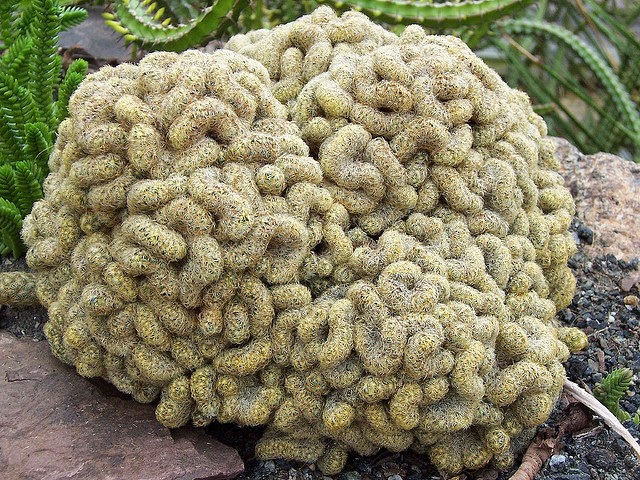The image captures a close-up of a peculiar mound of yellowish, brown-haired caterpillars tightly curled up and piled on top of each other, resembling a brain-like structure. They are nestled between two flat, large rocks—one reddish with gray spots on the left and a whitish rock with gray spots on the right. In the bottom right corner, black dirt scattered with pebbles and a branch can be seen, while the top left corner is adorned with several spiny, tentacle-like green plants. The overall scene suggests a rocky, desert-like environment where these caterpillars have gathered, possibly hinting at a natural assembly for either protection or transformation into cocoons.